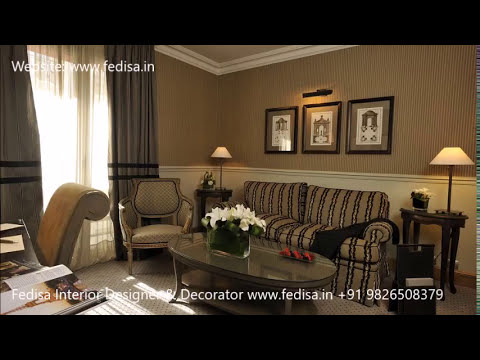The advertisement showcases a newly designed living room with a meticulous and modern interior. The space features a dual-toned wall, with the upper half in a dark beige and the lower half in light beige, separated by a white chair molding. The ceiling also boasts white crown molding. Dominating the right wall are three framed pictures, evenly spaced above a dark gray sofa with brown vertical stripes.

On either side of the sofa are wooden end tables, each adorned with a lamp featuring a white shade. An oval-shaped wooden coffee table stands in front of the sofa, topped with a basket of white flowers. A cushioned chair, upholstered on both the back and bottom, is positioned near the window on the left side. The window is dressed with white drapery flanked by gray curtains with black horizontal stripes.

Text above the room reads "Fedisa Interior Designer and Decorator" along with the website www.fedisa.in and the contact number +919-826-508-379, all left-aligned. The image is framed by a horizontal black bar at the top and bottom, adding a sleek finish to the advertisement.